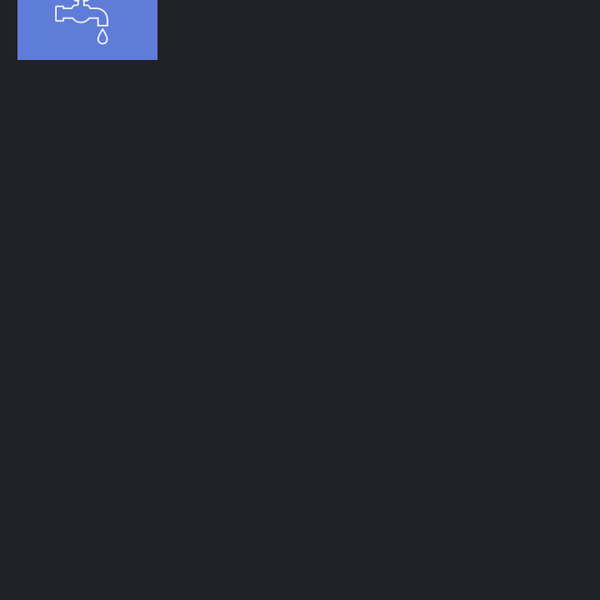The image is predominantly black, with what appears to be a slightly taller-than-wide square format. Positioned towards the upper left section, though not exactly in the corner, is a blue rectangle. This rectangle extends downward and features a white outline of a faucet—reminiscent of those typically attached to an exterior wall for hose connections. The faucet is depicted from a side profile, showing an incomplete outline of a droplet emerging from its spout. Notably, the top part of the faucet, including the handle, is partially cut off by the boundary of the blue rectangle, leaving only a minimal portion visible. The faucet icon is centrally aligned within the blue rectangle. The overall color scheme of the image comprises black, blue, and white, with the majority being black. No additional elements or background details are present in the image, leaving the outlined faucet as the sole focal point.